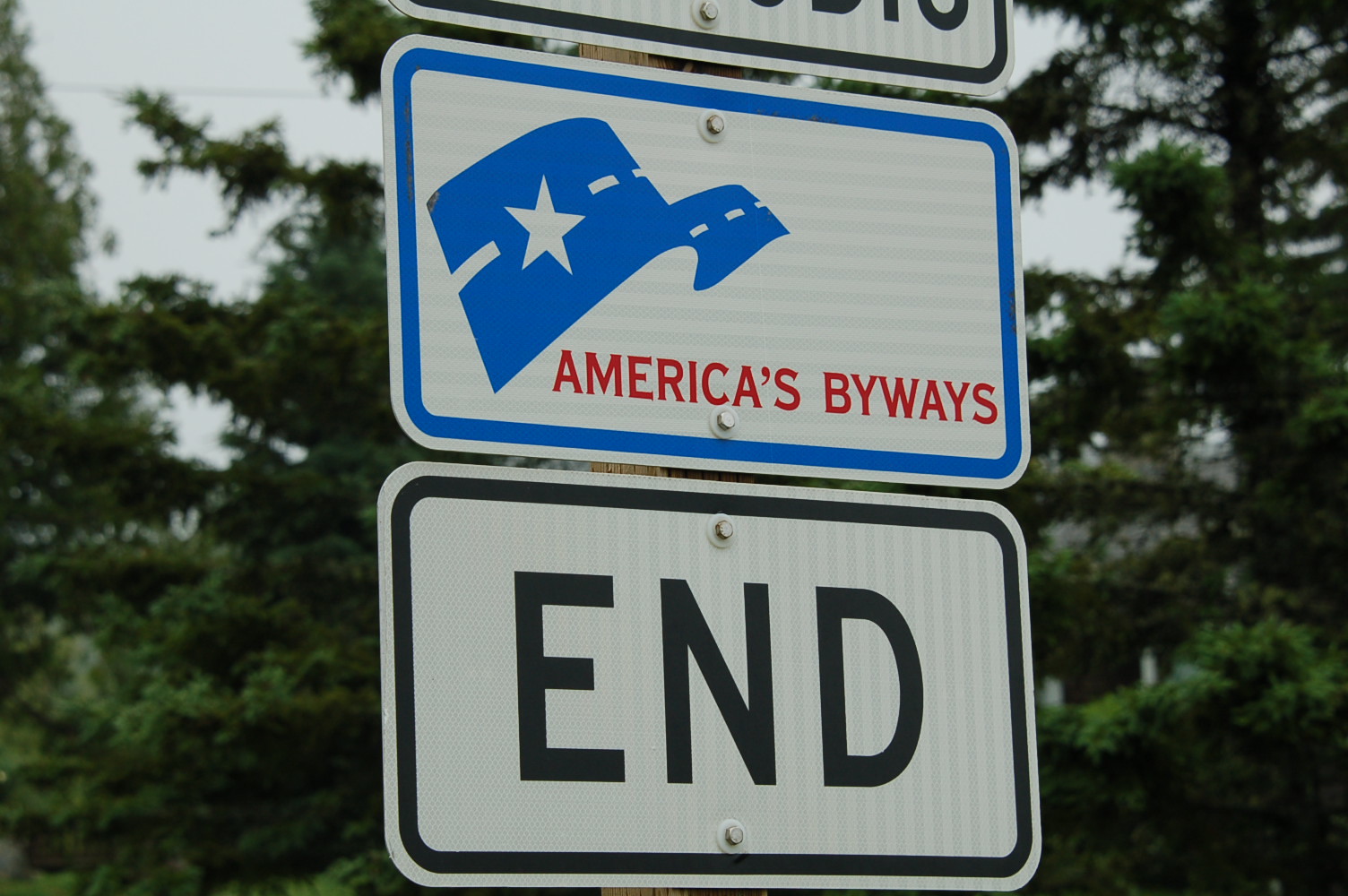The photograph features two prominent white street signs mounted on a brown wooden post, with the partial edge of an additional sign visible at the top. Both visible signs are secured with bolts at their top and bottom. The middle sign boasts a blue-bordered white background, with a blue graphic depicting a road with white dashed lines leading to a central white star. Below this graphic, red text declares "America's Byways," reflecting patriotic colors reminiscent of the American flag. The bottom sign is simpler, outlined with a black border and featuring bold black text that reads "END." Surrounding the signs, the backdrop showcases tall pine trees with lush green leaves set against a sky that shifts between blue and gray hues, suggesting a bright, yet not overly sunny, day. The overall scene captures the essence of an American roadway flanked by natural greenery.